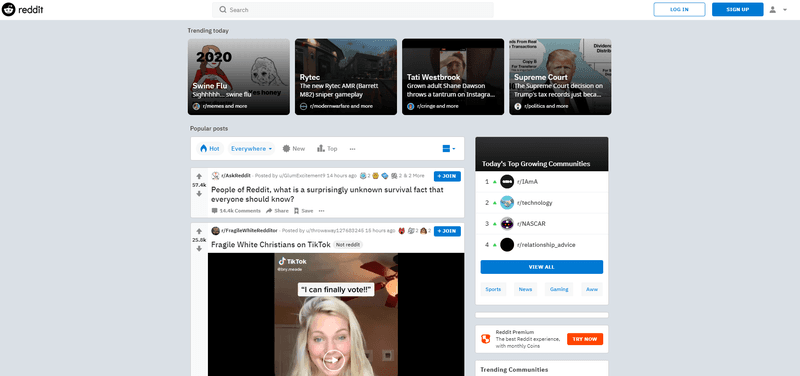This screenshot captures a desktop view of the modern Reddit interface. The top of the page features a navigation bar with a white background, stretching across the screen. On the left side of the bar, the Reddit logo appears inside a black circle, featuring the iconic white Snoo character. Next to it, "reddit" is displayed in black text. 

Centrally positioned in the bar is a grey search box, accompanied by a darker grey search icon and the word "Search" inside it. To the right, there are two buttons: one is a blue-outlined white box with blue text that reads "Sign In" or "Log In," and the other is a solid blue box with white text that says "Sign Up." Further to the right is the user icon followed by a dropdown arrow.

Below this navigation bar, the entire background of the screen is grey. A section titled "Trending Today" showcases four square tiles featuring trending news articles. The articles are about the Swine Flu, Ritech, Taddy Westbrook, and the Supreme Court, each represented by relevant images.

Under the trending section, a section for "Popular Posts" begins. The navigation options here include a white bar with "Hot" in blue text, a drop-down menu labeled "Everywhere," and grey text options for "New" and "Top." 

The first subreddit listed is r/AskReddit with a post titled, "People of Reddit, what is a surprisingly unknown survival fact that everyone should know?" This post includes a blue "Join" button. Below that is another thread, though the details are partly unreadable, the title "Fragile White Christians on TikTok," along with a clickable video.

On the right side of the screen, there is a black bar titled "Today's Top Growing Communities," listing subreddits such as IAMA, Technology, NASCAR, and Relationship Advice. This section includes a blue "View All" button, with further categorized grey boxes for Sports, News, Gaming, and All. At the bottom, an advertisement for Reddit Premium is displayed.